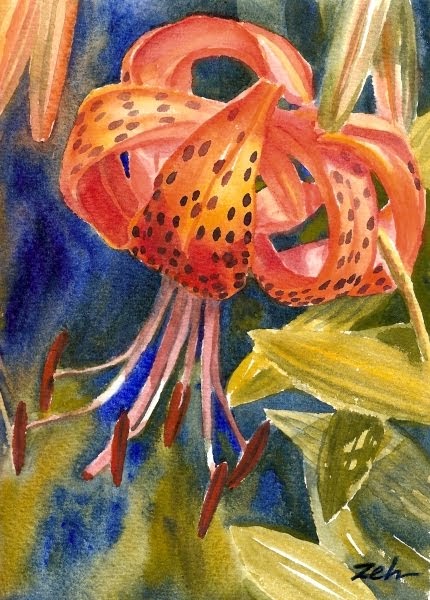The artwork depicts a single prominent flower resembling an iris, characterized by its downward-tilted petals that are primarily peach-like red with black speckles. The petals curve downward but then bend backward, creating an elegant and dynamic shape. Long stalks extend from the flower's center, fanning outward in a circular, implied motion, with brown, C-like appendages at the peaks. The background includes additional flowers and elements: purple flowers with brown tips grow beneath the central flower, while yellow-green bulb-shaped flowers extend from the right side towards the center. The scene is set against a vibrant backdrop featuring shades of blue and green, contributing to a lively and richly detailed composition. The painting includes signatures and markings; notably, the artist has signed their name "ZEH" in black in the lower right corner.